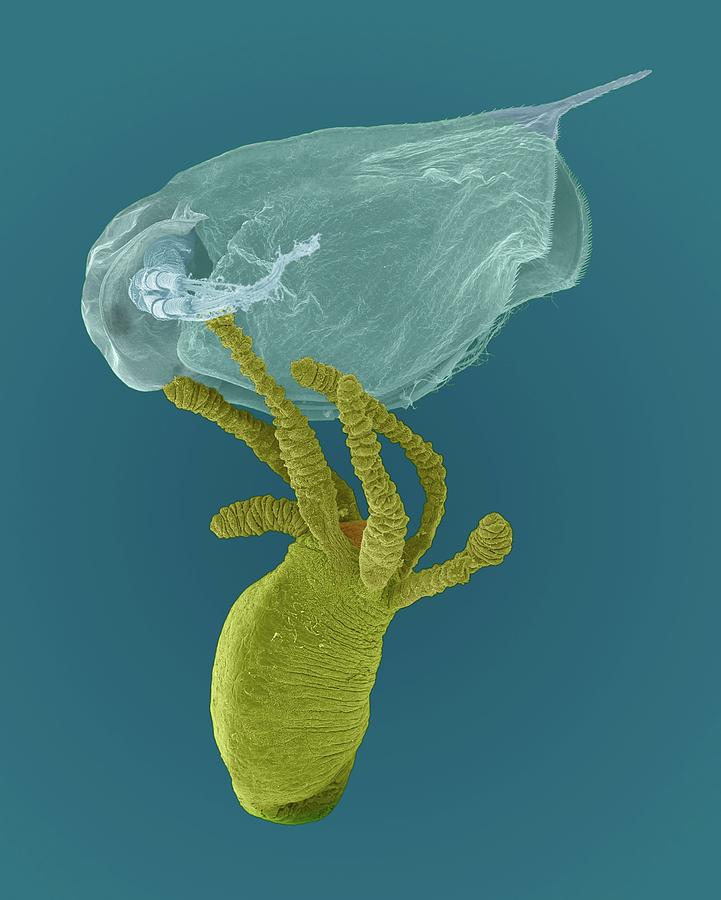In the image, we see a mesmerizing aquatic scene with a crystal-clear jellyfish, almost gossamer in its translucence, allowing a full view through its body. The jellyfish’s dome-like head, crowned with an intricate structure, is adorned with tentacles that unusually remain close to its body. Below the ethereal jellyfish, a striking green creature, resembling a six-armed squid with knobby, rough tentacles, appears to be engaging in a fierce struggle with the jellyfish.

The backdrop of this underwater tableau is a captivating bluish hue, adding a surreal element to the scene that blurs the lines between reality and art. This blue, though unnamed, is striking and draws the eye to the unusual pair of sea creatures. The complexity of the scene is further enhanced by additional forms; a vague suggestion of creatures that could be mistaken for spongy, nondescript sea urchins or upside-down yellow octopuses. Together, these elements hint at an intriguing underwater battle for dominance, set against a vividly colored marine backdrop.